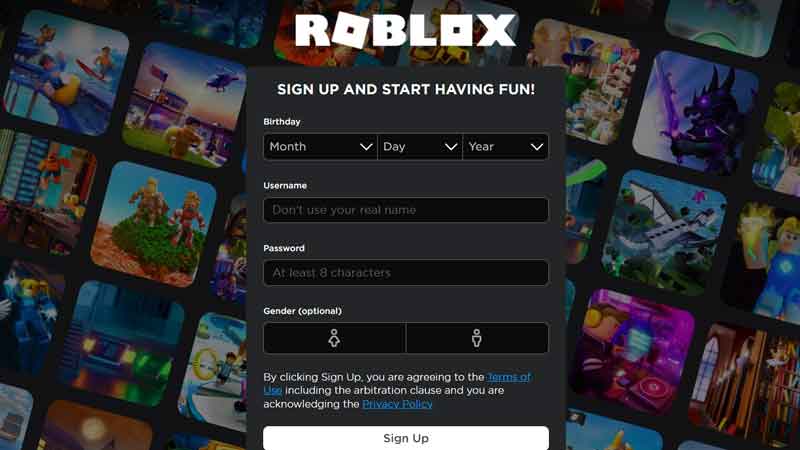The image is a screenshot from a website that appears to be the sign-up page for Roblox. The background displays various softly blurred squares, each filled with different video game graphics featuring various characters and settings on both the left and right sides.

At the top center of the image, "Roblox" is prominently displayed in bold, bubble letters. The first "O" in "Roblox" is slightly tilted upward. Directly below this, there is a light black square containing text. In white capital letters, it reads: "SIGN UP AND START HAVING FUN!" with an exclamation point at the end.

Further down, the form fields for the sign-up process are visible. The first section is labeled "Birthday" and includes three drop-down menus for selecting the month, day, and year. Below that is a field labeled "Username" with a note advising users not to use their real name. Following this is a "Password" field with instructions that the password must be at least eight characters long, where the "eight" is written as a numeral.

The form continues with a "Gender" section marked as optional, where users can select "Girl" or "Boy." At the bottom of the form, there is a disclaimer stating that by clicking "Sign Up," users agree to the terms of use (which is a hyperlink and includes an arbitration clause) and acknowledge the privacy policy (also a hyperlink).

Finally, there is a large "Sign Up" button set against a white background at the very bottom.